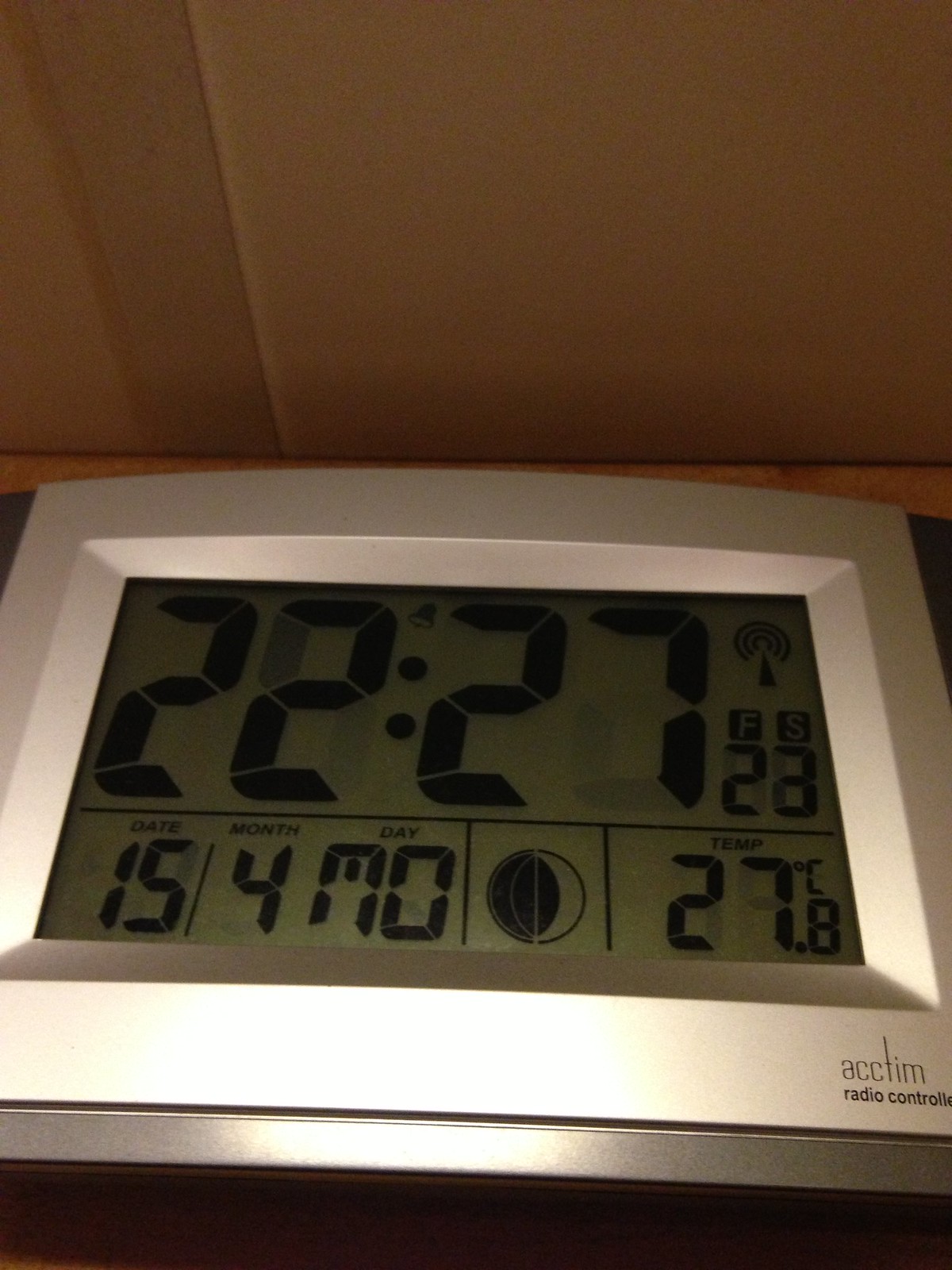This is a detailed photograph of a digital calendar clock, specifically an ACCTIM brand model, identifiable by the logo printed on the device. The clock is radio-controlled, as indicated directly below the brand name. The digital display features a grayish-greenish background and is divided into several informative sections.

At the top of the display, the time is shown in military format, reading 22:27, with the seconds counter adjacent, currently at 23 seconds. Below the time, the date is displayed as the 15th of April, alongside a visual representation of the moon phase, which appears to be a crescent moon, approximately a quarter full. Additionally, the temperature is indicated in Celsius, showing a reading of 27.8°C.

The entire digital display is encompassed by a thick, chrome or silver frame, adding a touch of modernity and robustness to the device. The clock is situated on what appears to be a wooden table, cabinet, or dresser. The surrounding room provides a subtle backdrop with walls painted in a light brown or dark tan color, enhancing the earthy and warm atmosphere of the setting.